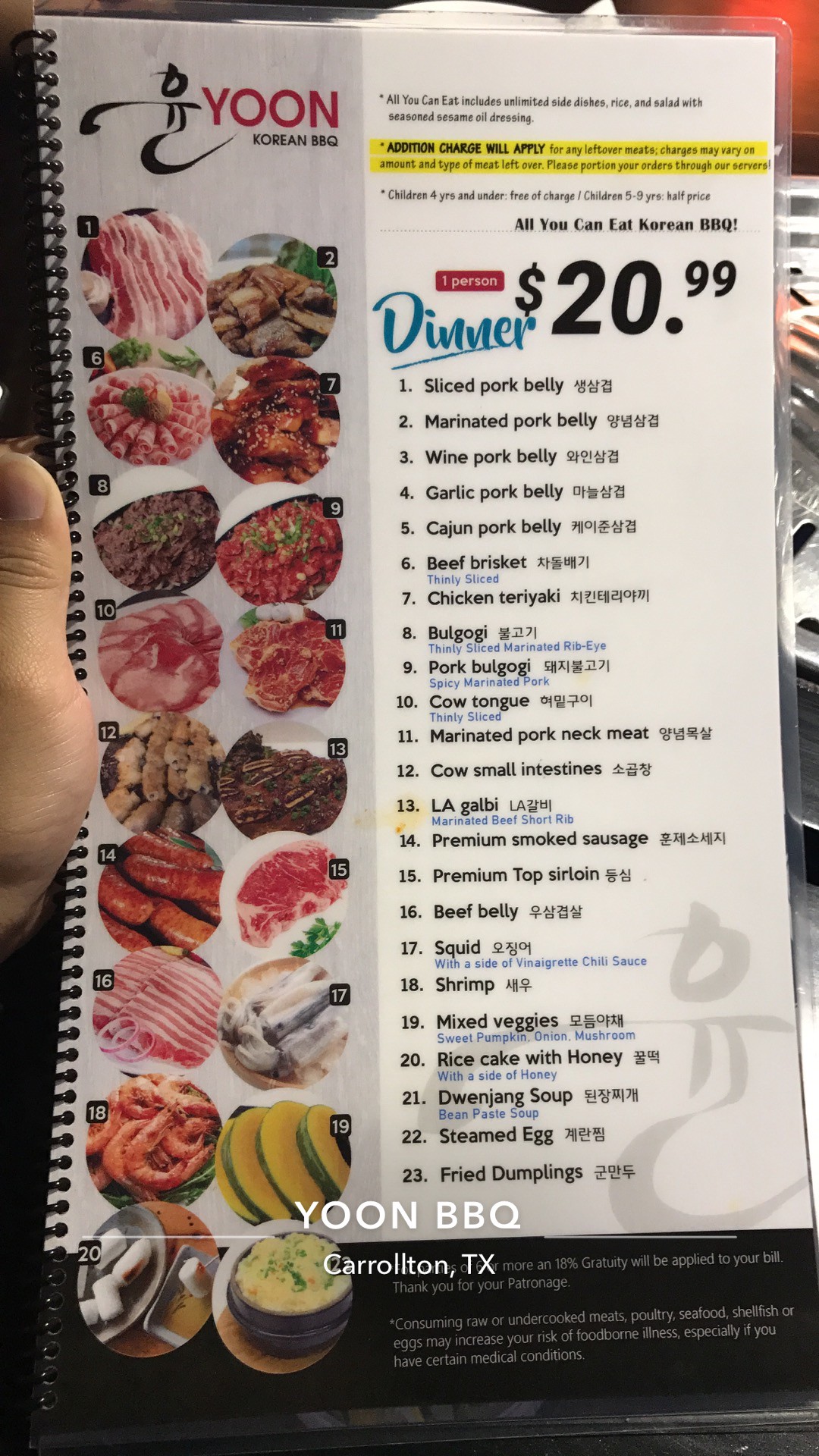This photograph displays a centrally positioned restaurant menu for Yoon Korean BBQ, spotlighting their dinner offerings priced at $20.99. The menu, covered in text listing various entrées, includes dishes such as bulgogi, beef brisket, Cajun pork belly, sliced pork belly, shrimp, squid, and premium top sirloin. A thumb is visible on the left side, holding the menu in place. A watermark at the bottom of the image, reading "Yoon BBQ Carrollton Texas," suggests the photo was taken on Instagram or Snapchat. The background hints at a restaurant table setting, though it remains largely out of focus.